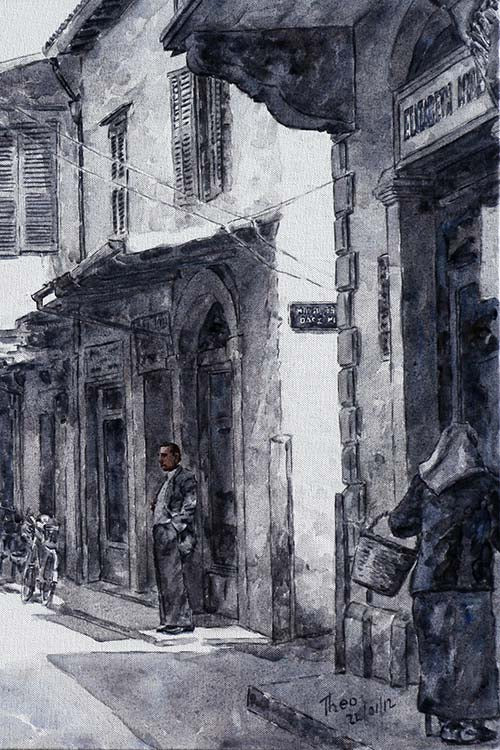This detailed, watercolor-style painting by Theo from 2012 captures a street scene characterized by shades of black, white, and gray, with subtle hints of color. The scene is depicted in a vertical rectangle format, focusing on an array of storefronts and their architectural details. On the right side, a two-story stone and brick building with a large doorway draws immediate attention. An elderly woman, adorned with a small scarf on her head and a long, dark outfit, steps through the doorway carrying a basket over her left arm. Above the door, partially obscured by a roof support, is a sign that reads "Elizabeth."

Adjacent to this building, after a small alleyway, lies a second structure with an arched doorway and large window. Underneath an awning, a man dressed in a suit stands outside, his left hand casually placed in his pocket, and his brownish face turned toward the street. Further down the road, a bicycle rests against the façade of a barely visible third building. Above, the upper stories reveal window shutters, adding to the historic charm of the buildings.

The painting also includes various illegible signs that seem to indicate business or street names. The artist’s signature is located in the lower right-hand corner, subtly completing this evocative scene of everyday life.